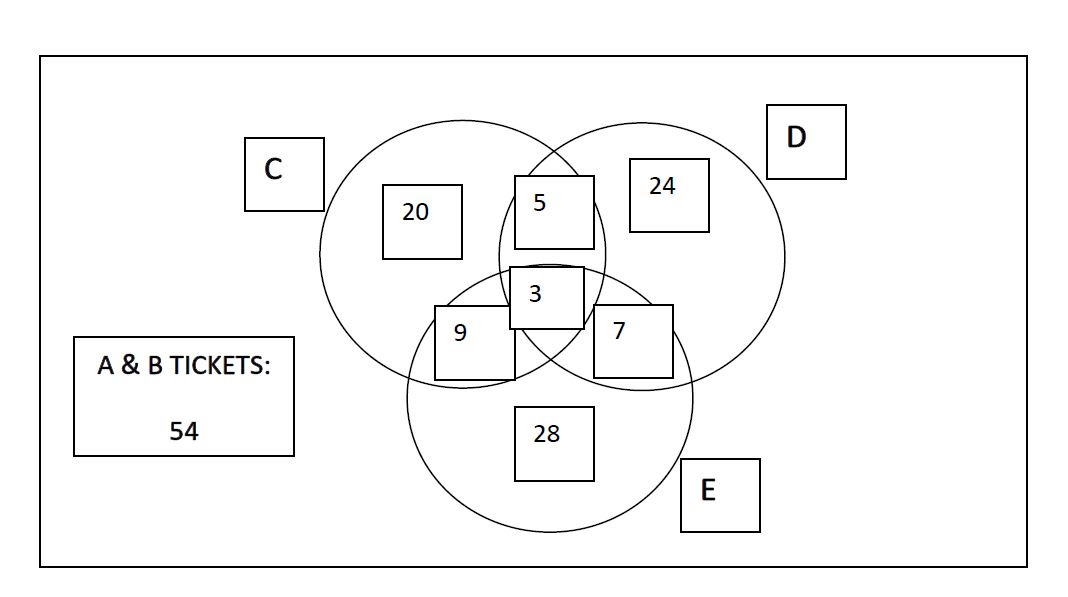The image is a hand-drawn Venn diagram consisting of three intersecting circles, labeled C, D, and E, positioned in the center. 

- **Circle C** (leftmost):
  - Contains a small rectangle with the number "20".
- **Circle D** (right of Circle C):
  - Contains a black rectangle with the number "24".
  - The intersecting area between Circle C and Circle D features a black rectangle with the number "5".
- **Circle E** (below Circles C and D):
  - Contains the number "28" on its own.
  - The intersection of Circles C, D, and E has a square bearing the number "3".
  - The overlap between Circle C and Circle E contains a square with the number "9".
  - The overlap between Circle D and Circle E has a square labeled with the number "7".

To the left of these circles, there is a separate rectangle labeled "A and B tickets: 54". The entire drawing is done in black ink on a white background.